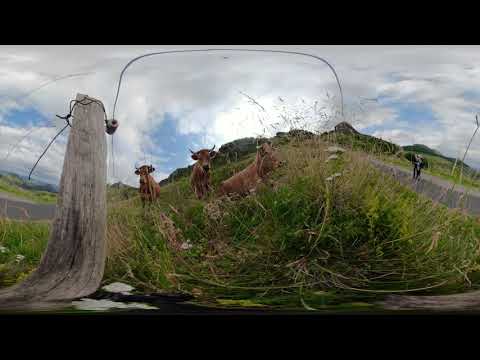In this outdoors daytime photograph, three brown cows, each with short white horns, are captured in a field of unkempt, tall green grass. They are all looking towards the camera, with one on the right partially hidden by the grass and the other two clearly visible. Beside the cows, a wooden post or tree stump is present on the left. The field is outlined by a wooden fence and dense, random weeds. In the background, there is an asphalt road with a person dressed in dark clothing walking on it, further set against a backdrop of rolling green hills and dark green tree lines. Above, the sky is mostly cloudy with light gray and white clouds, though patches of blue can be seen through the gaps. The overall scene portrays a peaceful rural landscape with vast and vivid natural details.